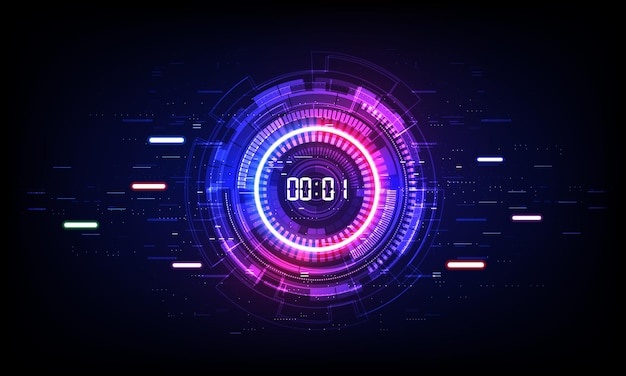The image features a rectangular display, approximately four inches wide and three inches high, with a predominantly black background. At the center of the image is a high-tech, sci-fi-inspired countdown clock, stylized with a circular arrangement of lights and lines. The clock displays "00:01" in white digital print, indicating one second left. Surrounding the numbers is a solid white circle, beyond which vibrant colors of reds, dark blues, and light blues radiate outward. These colors transition into purples and pinks at certain points, creating a visually striking gradient. The innermost circle, roughly an inch in diameter, transitions into lines and dots of color—orange, white, and green—that extend towards the image's edges. The outermost areas are filled with long horizontal lines and smaller dots, which gradually fade into the black backdrop. The design evokes a futuristic feel, reminiscent of scanning devices in sci-fi movies like Tron, with intricate patterns and illuminated details amplifying its high-tech appearance.